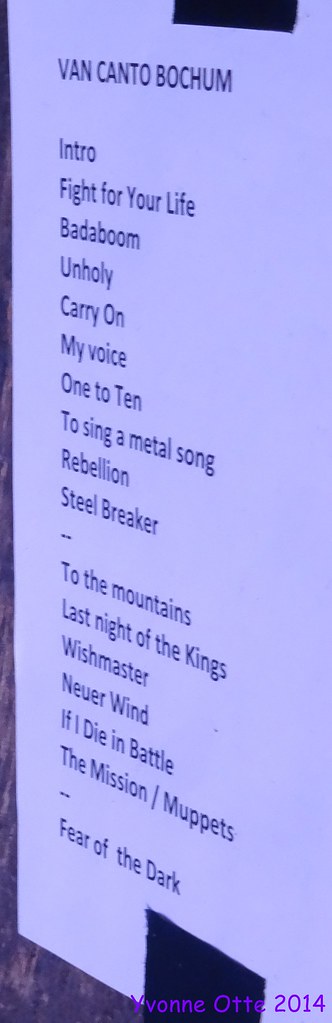In this image, a lightly purple-tinted white piece of paper, approximately three to four feet tall, occupies the center of the frame, dominating the entire photo. The paper is fixed to a wall or post, possibly outdoors, although the background is only partially visible. The text on the paper appears to be a list, featuring various titles that suggest songs, stories, or announcements. The titles include: "Ven canto bocum, intro, fight for your life, badum, unholy, carry on, my boys, 1 to 10, to sing a metal song, rebellion, steel breaker, to the mountains, last night of the kings, wish master, newer wind, if I die in battle, the mission muppets, and fear of the dark." The sign's inscription ends with the notation "Yvan Ott 2014" at the bottom, hinting at an event or collection by this individual. The image features various colors, prominently white, black, purple, and brown, with the large, detailed text-centered sign as the main focal point.